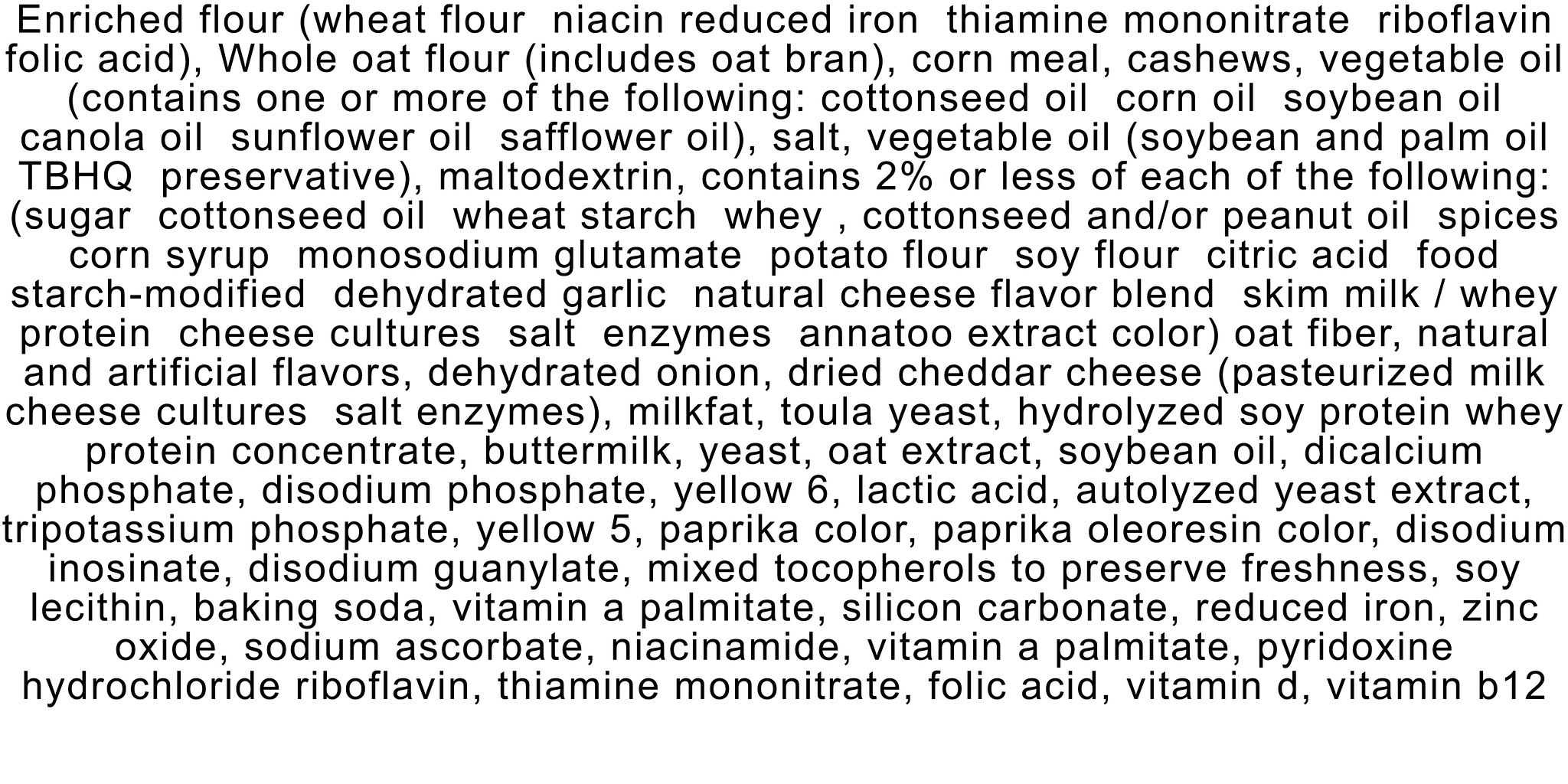The image displays a detailed, multi-ingredient label in black text on a white background. The label enumerates over 50 ingredients, including enriched and wheat flours, niacin, reduced iron, thiamine mononitrate, riboflavin, folic acid, whole wheat, and whole oat flour. It also mentions cornmeal, cashews, various vegetable oils (cottonseed, corn, soybean, canola, sunflower), TBHQ preservative, and maltodextrin. Minor components constituting 2% or less include sugar, wheat starch whey, spices, citric acid, dehydrated garlic, cheese flavor blend, oat fiber, milk fat, yeast, soy protein, and buttermilk. No brand names or nutritional information are presented, leaving the actual food product unidentified. The extensive list, noted to have a grayish tone, hints at a highly processed item, possibly baked or snack-related.